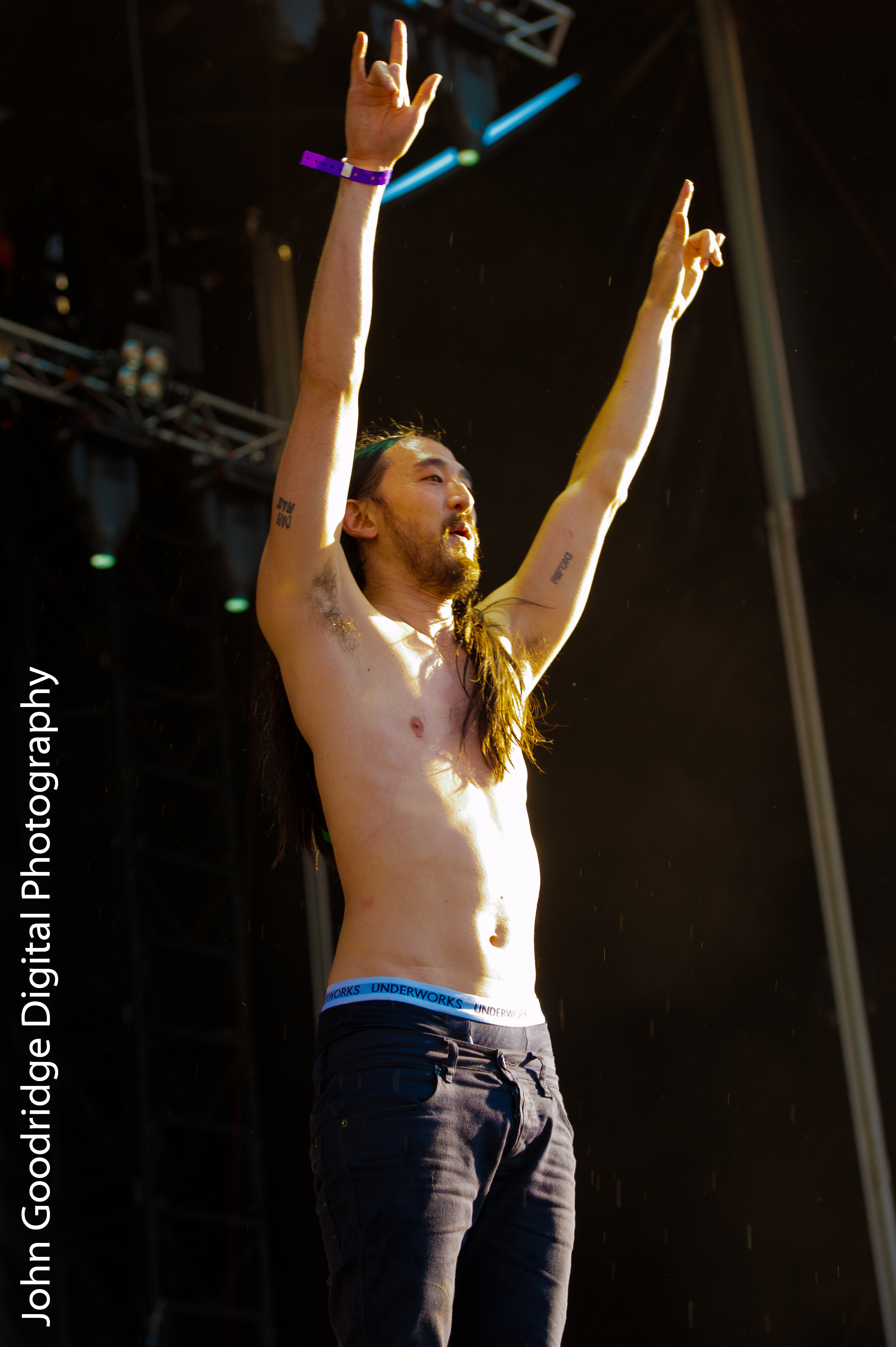A vertically oriented rectangular photograph captures a shirtless man on stage, exuding confidence and charisma. His attire includes black jeans and partially visible underwear with a white waistband branded "Underworks," and hints of black beneath. The man, a slender figure, stands with both arms raised in front of him, forming peace signs with his hands. His long brown hair is tied in a ponytail draped over his left shoulder, complementing his brown beard and mustache. Small tattoos are scattered across his arms, adding unique details to his appearance. Behind him, a dark stage background is punctuated by four spotlights on the upper left, mounted on bars, and symmetrical blue lights flanking the upper middle section. The man's open mouth suggests he is mid-speech or performance, adding dynamic energy to the scene. Along the left edge of the image, the vertical text "John Goodridge Digital Photography" is elegantly printed in white letters, marking the artist's credit.